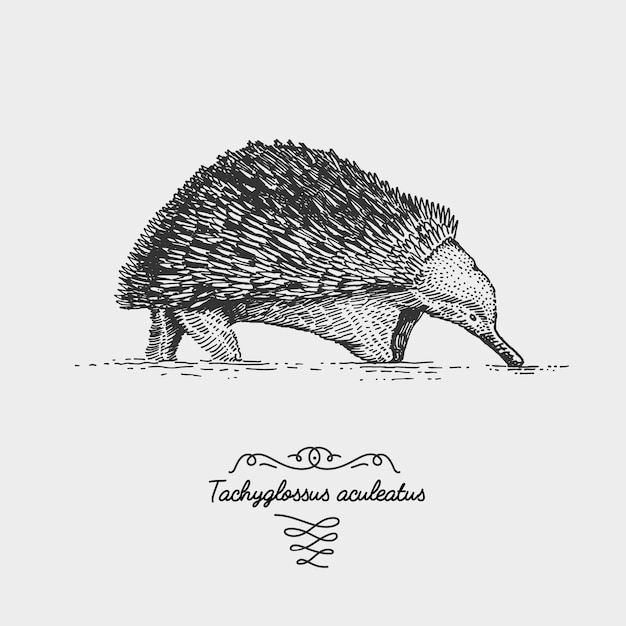The image features a detailed sketch of an animal identified as Tachyglossus aculeatus. The background of the artwork is a light gray color, creating a neutral backdrop that accentuates the intricate lines of the drawing. Rendered in fine tip marker or pen, the animal resembles a hybrid of a hedgehog and an anteater, possibly even a platypus with a spiky back. The creature's oval-shaped, dome-like back is covered with long, spiky quills. Its head, textured with spots and shaded areas, extends into a long black nose, indicative of an anteater. The animal has a visible black eye and short, stubby legs adorned with fine lines mimicking a hairy texture. Underneath the sketch, there is text that reads "Tachyglossus aculeatus," accompanied by an ornate design of swirling black lines, adding an artistic flourish to the scientific illustration.